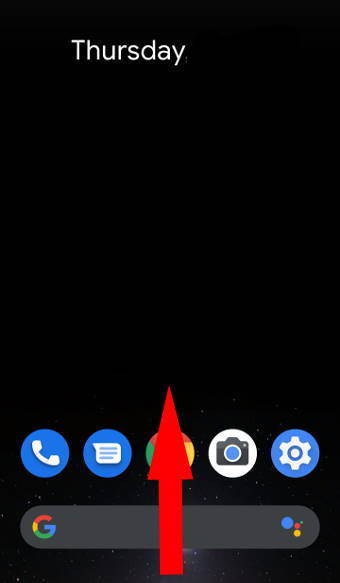This image is a detailed screenshot of a smartphone screen. On the top portion of the screen, the word "Thursday" is clearly displayed, signifying the current day. The background is predominantly black, offering minimal content, making it challenging to identify the specific app at first glance. However, the presence of what resembles a Chrome logo suggests it could be an iteration of the Chrome browser.

At the bottom of the screen, a menu bar features five distinct icons in the following order from left to right: a phone, a text message, a possible Chrome logo, a camera, and settings. Directly below this menu bar, at the very bottom of the screen, lies a Google search bar prominently featuring the Google logo.

Enhancing the overall layout of the screenshot is a red arrow, originating from the bottom of the screen and extending upward to about one-third of the way up the image. This arrow points towards the top of the screen, with its arrowhead almost directly over the suspected Chrome logo, creating a visual overlap and contributing to the initial uncertainty regarding the app's identity.